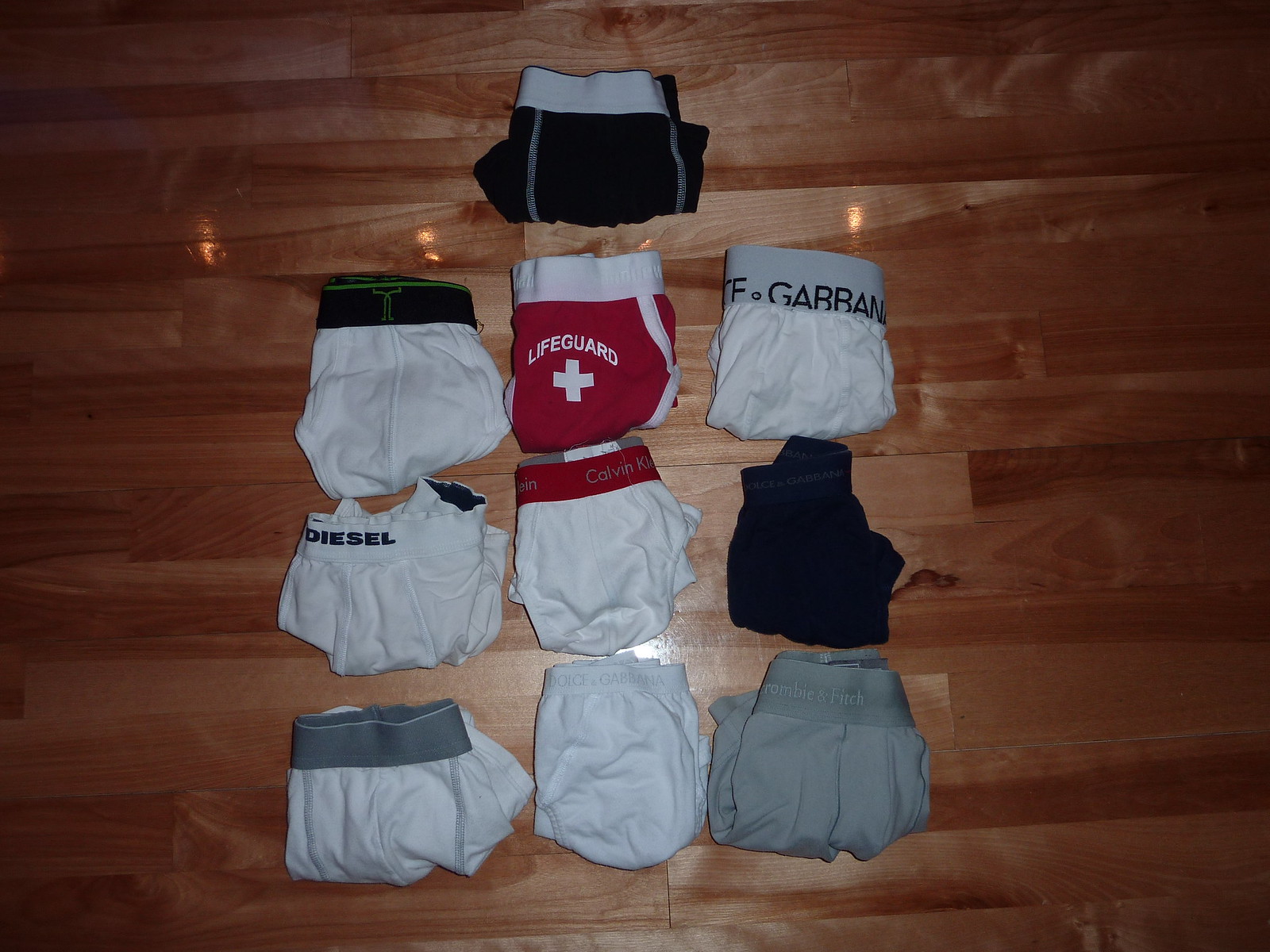This color photograph captures an array of eleven pairs of men's underwear, all neatly folded and displayed on a polished, light brown wood floor adorned with dark brown streaks and visible knots. The surface of the floor is reflective, with light reflections visible at the top and bottom center of the image. The underwear, which are organized in rows of three with one pair alone at the top, feature a variety of brands and designs. The topmost pair is black with a white waistband accented by two gray stripes. Below it is a pair with a black band and lime green accents, followed by red underwear with white trims and the word "Lifeguard" in bold red letters, paired with a white cross. Another noteworthy pair has a white band reading "Dolce & Gabbana," partially visible, next to a pair with a white band and the name "Diesel" in dark blue letters. Additionally, there's white underwear with a red band from Calvin Klein, gray and black pairs, and an Abercrombie & Fitch pair in dark gray with a silver band. The diverse assortment of designs and brand names, such as Calvin Klein and Diesel, suggests these might either be new purchases or items being sold.